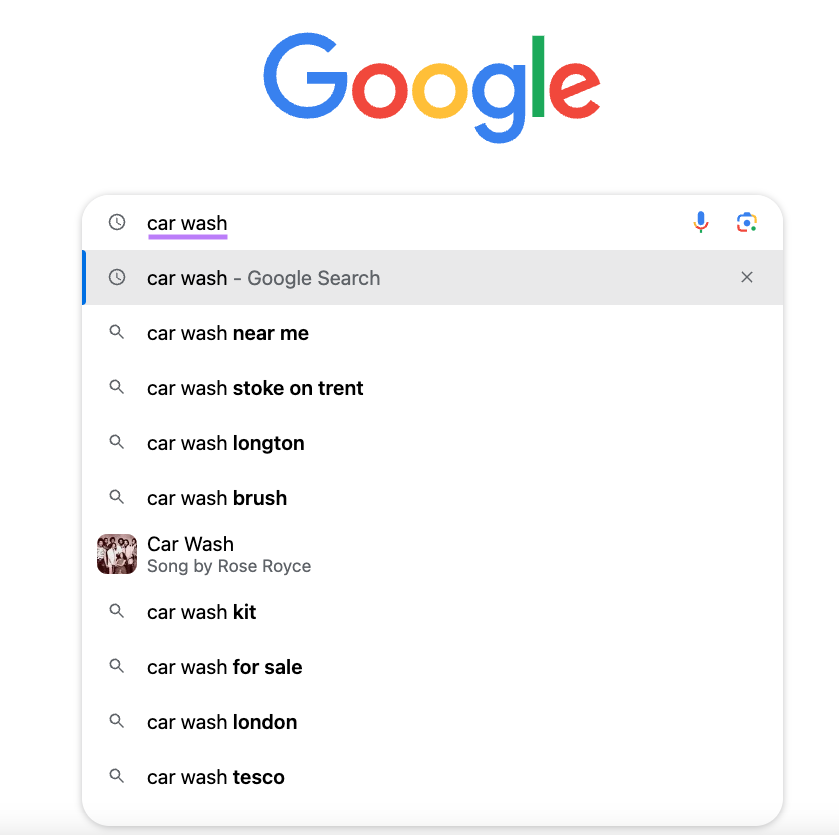The image is a screenshot of the Google website displaying search results for the term "car wash." The screenshot is approximately square-shaped, featuring a predominantly white background with black text. A colorful Google logo, with letters in blue, red, yellow, blue, green, and red (from left to right), is prominently centered at the top of the page. Directly beneath the logo is the search bar, where "car wash" has been entered and underlined with a purple line.

Under the search bar, a drop-down menu appears, showing Google's suggested search options. The top suggestion, highlighted in gray with a vertical blue bar on the left, is "car wash - Google Search." Additional suggestions include "car wash near me," "car wash Stoke-on-Trent," "car wash Longton," "car wash brush," and "car wash song by Rose Royce," which is accompanied by a small thumbnail image of a group of people in black and white. Further suggestions listed are "car wash kit," "car wash for sale," "car wash London," and "car wash Tesco."